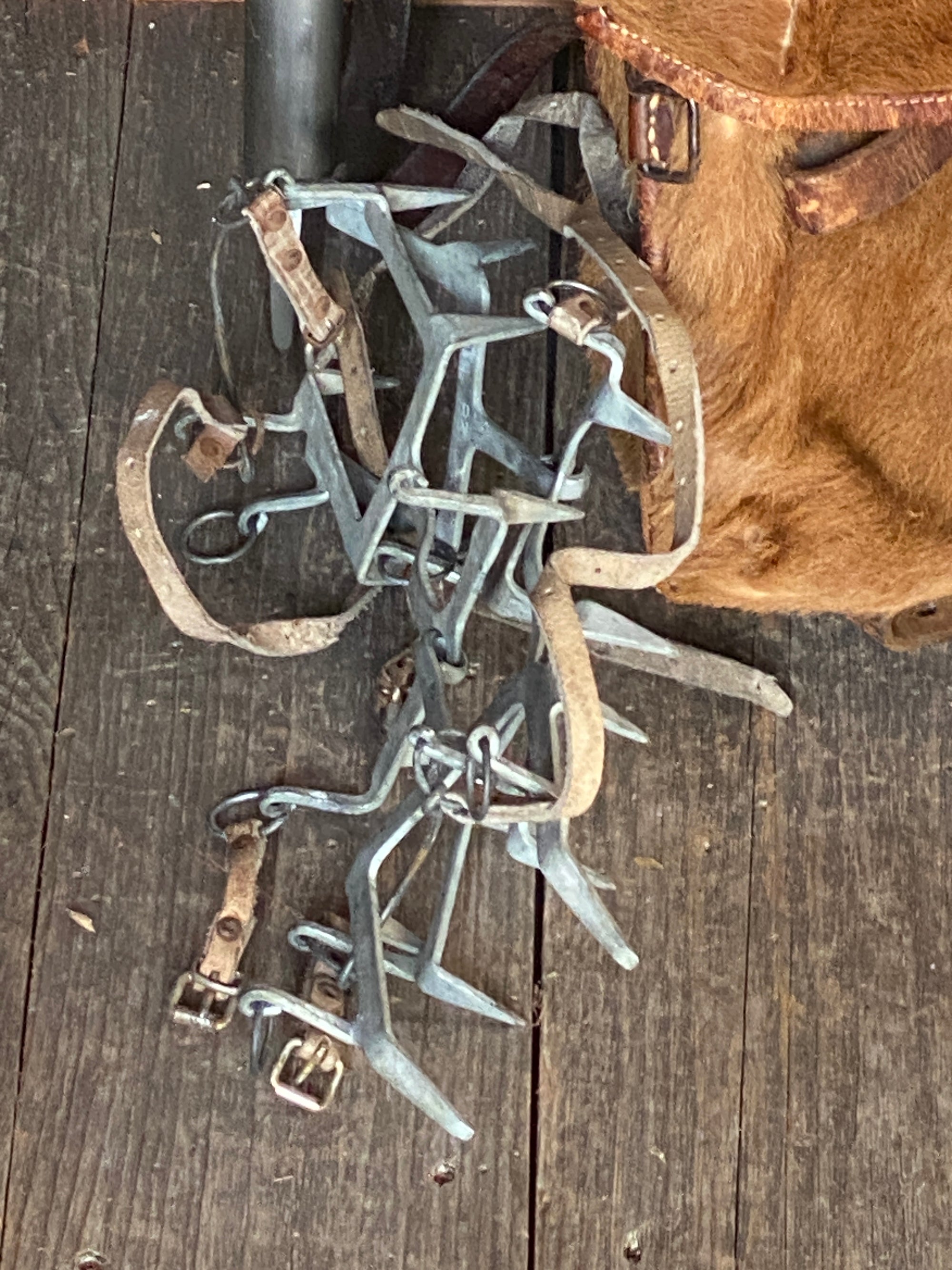The image portrays a rustic western scene, centered on a weathered wooden floor marked by cracks and nail indentations. Piled haphazardly in the middle are several pieces of horse tack, including four tangled horse harnesses with sharp metal prongs and rings, all intertwined with brown leather straps. In the bottom left corner is a string of silver, spike-laden spurs, while in the upper right corner rests a cowhide bag or animal hide sack, distinguished by its fur and a single visible eye, adding a touch of rustic authenticity to the scene.